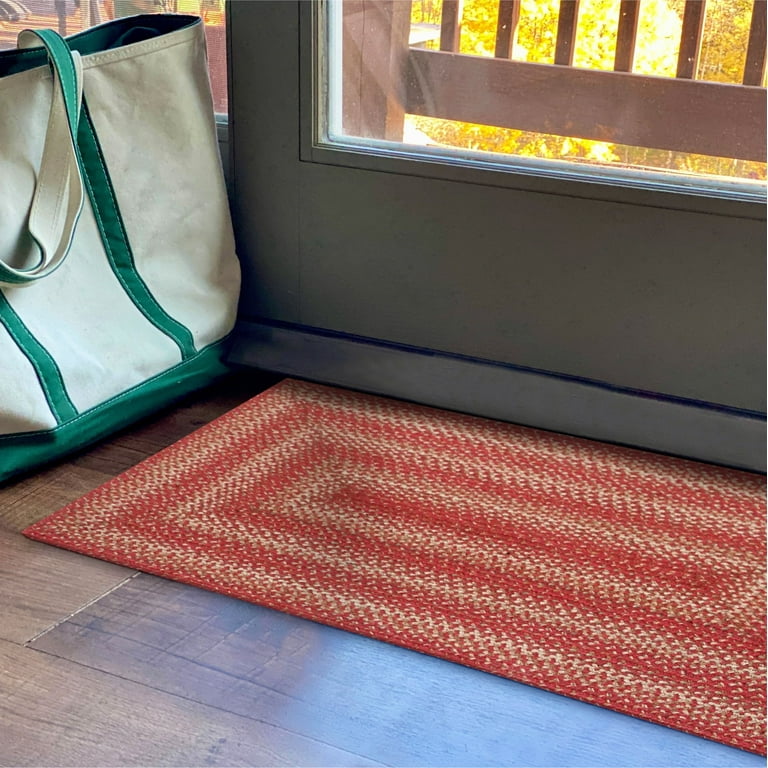In the center of the image is a small, handmade, rectangular rug with a pattern of concentric rectangles. The innermost rectangle is a thin red line, followed by alternating larger rectangles of a cream color and red, or possibly various shades of orange. The rug is placed on a wooden plank floor in front of a sliding glass door. Sunlight streams through the door, illuminating the scene. Outside the door, part of a deck or patio and a wooden fence are visible, with glimpses of trees in the background. To the left of the rug, a canvas tote bag with white and green stripes and green handles adds a touch of casual charm to the setting.